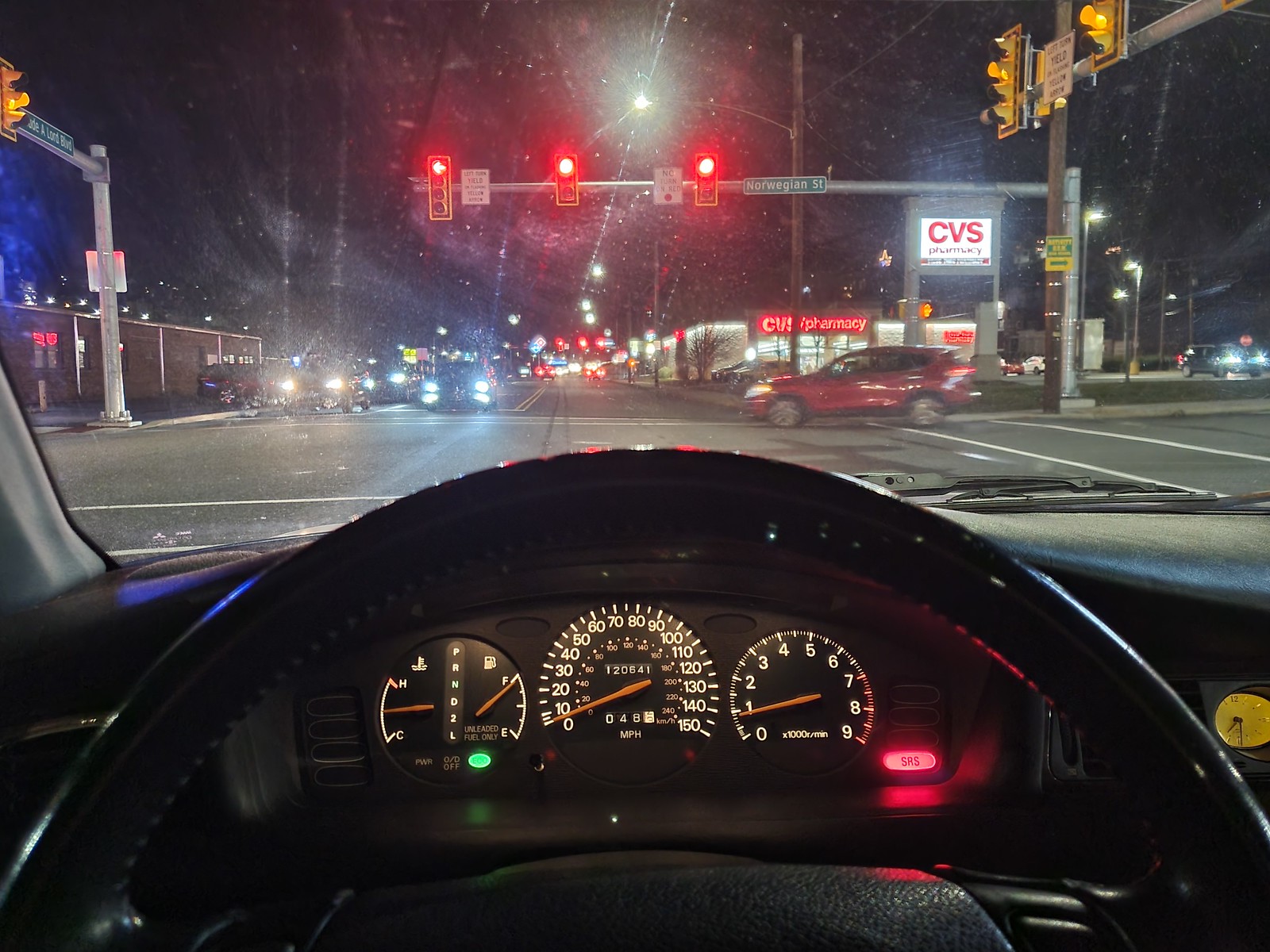Captured from the driver's seat inside a car, this nighttime photograph showcases an urban street scene framed by the windshield. The vehicle is paused at a red light, underscored by the glow of its own black and white-lit dashboard. In the foreground, a red car approaches from the right, preparing to cross in front of the stopped vehicle. Distant streetlights and traffic signals, all glowing red, contribute to the ambient cityscape, while the unmistakable storefront of a CVS pharmacy punctuates the right side of the frame. The car's interior is bathed in subdued lighting, with illuminated gauges standing out against the black material. Notably, a red SRS indicator light is visible on the dashboard's right side, and a smaller, ambiguous green light glimmers on the left.